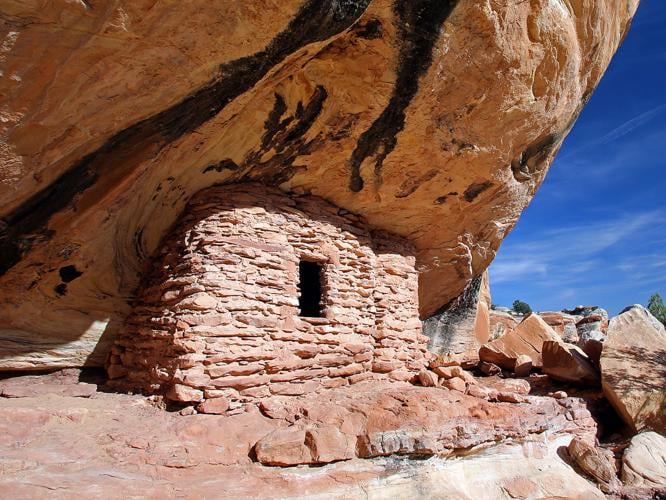The image depicts a makeshift shelter ingeniously constructed from reddish desert rocks, nestled under a dominating cliff overhang on a mountainous terrain. The shelter features a small window and is crafted from the same red rock material that characterizes the surrounding environment. In the backdrop, a striking blue sky with wisps of white clouds stretches across, providing a vivid contrast to the rugged landscape. Larger rocks populate the right side of the photo, introducing shades of darker brown and black. Two green trees are faintly visible in the background, adding a touch of greenery to the otherwise arid scene. The overall setting is brightly lit, accentuating the unique textures and hues of the rock formation, and imbuing the scene with a slightly mysterious allure.